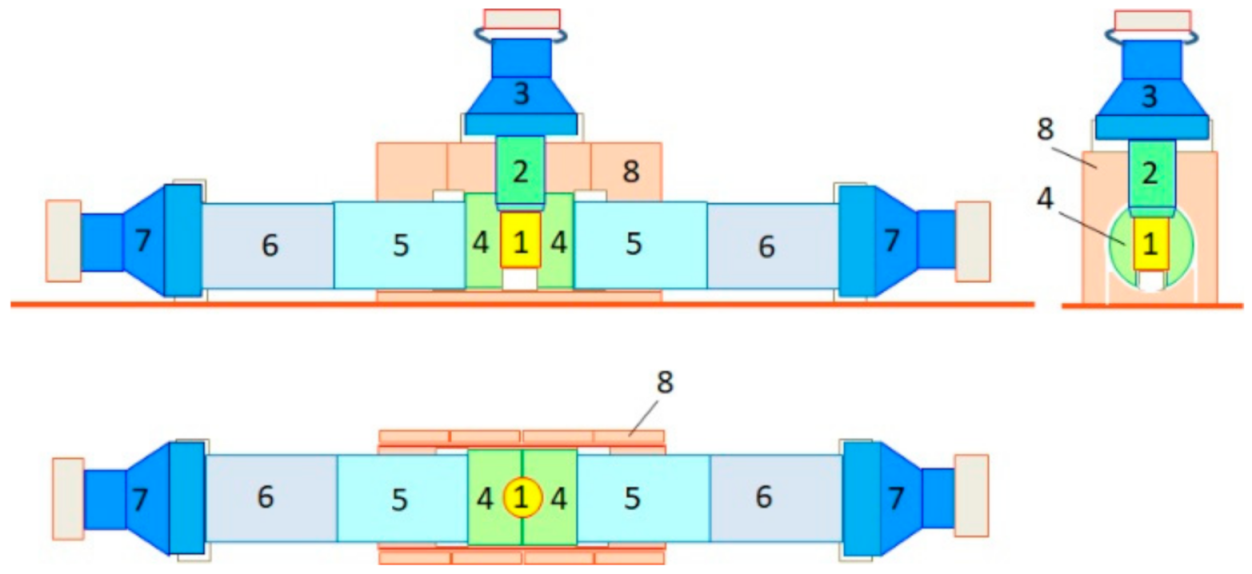The image displays a detailed, unlabeled mechanical diagram, possibly from a schematic or a textbook, depicting the breakdown of a complex assembly. The primary structure resembles a long exhaust system or piping, characterized by identical cylindrical components with a vertical offset, presented both in stacked views and in a right-side profile. The assembly consists of various shapes, including rectangles, trapezoids, and circles, all colored in shades of gray, light blue, dark blue, sky blue, green, yellow, purple, and orange. Numerical labels (ranging from 1 to 8) are marked in different colors throughout the diagram, though there is no legend to define these numbers. Prominently, the number 8 and 4 are repeatedly referenced with arrows. The top section features a trapezoidal shape and multiple colored sections including an orange rectangle and a green protrusion. The bottom section mirrors the cylinder but omits the trapezoid and green rectangle. On the top right, a side profile indicates additional rectangular components and overlapping shapes. The diagrams include a series of colored blocks and shapes that correspond to specific numbers, potentially indicating parts or connections within the assembly.